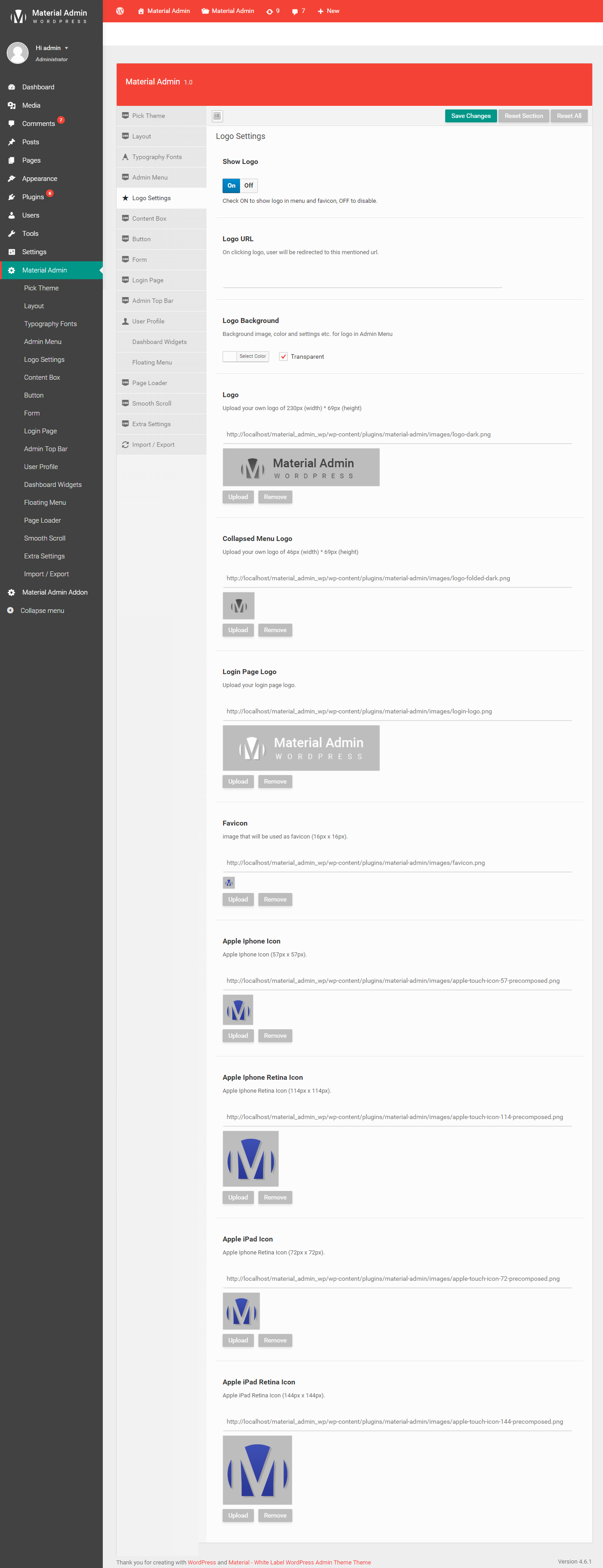This image depicts a snapshot of a programming application displayed on a computer screen, taken from a distance which makes the text somewhat difficult to discern. On the left side of the interface, there's a prominent vertical black sidebar. At the top of this sidebar, a logo featuring a black 'M' within a white circle is visible. Just to the right of this logo, the text "Material Admin" appears multiple times, suggesting that this is the name of the application.

Beneath the logo, there's an avatar placeholder intended for a user profile picture. Further down the sidebar, there are several navigation links, though their labels are not entirely readable due to the distance. However, one of the links is clearly labeled "Menu," and two others are marked with red dots.

On the right side of the screen, horizontal red bars are evident at the top, possibly indicating active selections or notifications. When a link is clicked, it appears to redirect to another page where the navigation links are then displayed within a vertical gray bar. The main content area, positioned to the right of these bars, features a white background with additional navigation options, allowing deeper access into the application's settings.